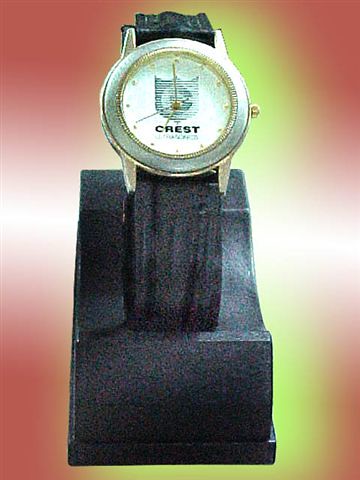This photograph elegantly captures a man's dress watch in portrait mode, set against a rose-orange background that exudes a warm, inviting glow. The backdrop features subtle white reflections and a radiant yellow light encircling the black rectangular base that supports the timepiece. Positioned centrally in the image, the watch is displayed vertically, showcasing its sophisticated features. The black leather band seamlessly complements the watch's gold-colored bezel and numerals. The watch face is strikingly white, inscribed with the word "Crest" at the bottom, and adorned with a central shield emblem. Time is indicated by gold hands pointing precisely to seven o'clock, further enhancing the watch's classic elegance.